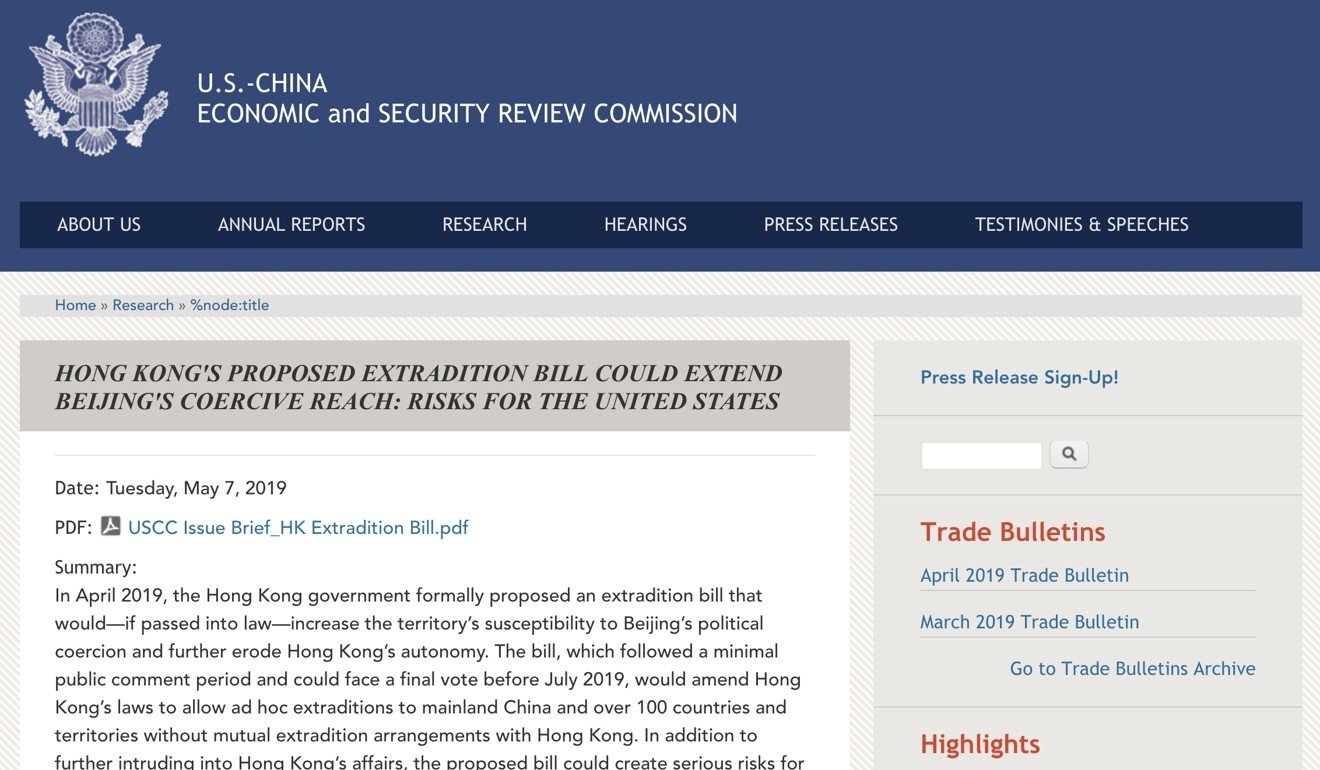This image is a screenshot from the website of the US-China Economic and Security Review Commission. At the upper left-hand corner, there is an emblematic black and white eagle holding various items and flowers, including a prominent sunflower, in its lower feet. This emblem is set within a grayish-blue rectangular banner at the top of the page.

Below this banner, there is a long, skinny, dark blue rectangle featuring navigation options in white text. From left to right, these options are labeled: "About Us," "Annual Reports," "Research," "Hearings," "Press Releases," and "Testimonies and Speeches."

Following this section, the page's breadcrumb navigation indicates the user has navigated from "Home" to "Research" and then to an undefined node titled "Hong Kong's Proposed Extradition Bill Could Extend Beijing's Coercive Reach: Risks for the United States." An introductory paragraph beneath this title begins with a reference to April 2019, summarizing the content that discusses the implications of Hong Kong's proposed extradition bill on U.S. interests.